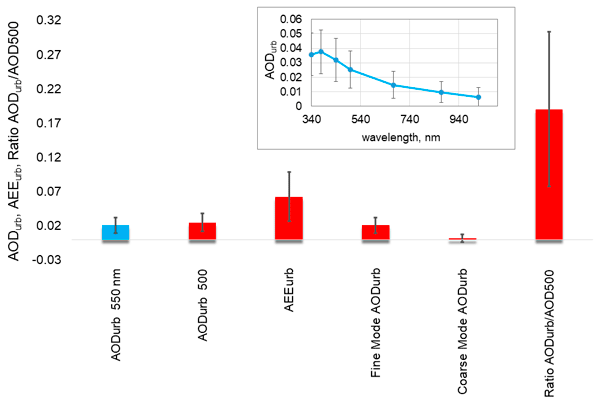The image features a detailed bar chart with vertical red and blue bars of varying heights, ranging from approximately 0.01 to 0.32 on the y-axis. The y-axis displays values starting from -0.03 to 0.32. The x-axis categorizes the bars with acronyms such as AOD, AEE, Fine Mode AOD, Coarse Mode AOD, and Ratio AOD, specifically labeled with measurements like 550 and 500 nanometers. Each labeled bar represents a specific set of data: for instance, the AOD URB 550 nanometers bar rises to about 0.02, while the Ratio AOD URB/AOD 500 bar peaks at nearly 0.17.

Embedded in the upper right corner of the main bar chart is a smaller, related line chart, which details wavelengths in nanometers ranging from 340 to 940 nm. In this line chart, a blue line ascends slightly before gradually descending, representing the variation of a particular dataset over the range of wavelengths. The accompanying numbers on the left-hand side of this inset graph span from 0.06 down to 0. The overall layout appears meticulous, although it lacks explicit titles for both the x and y axes.